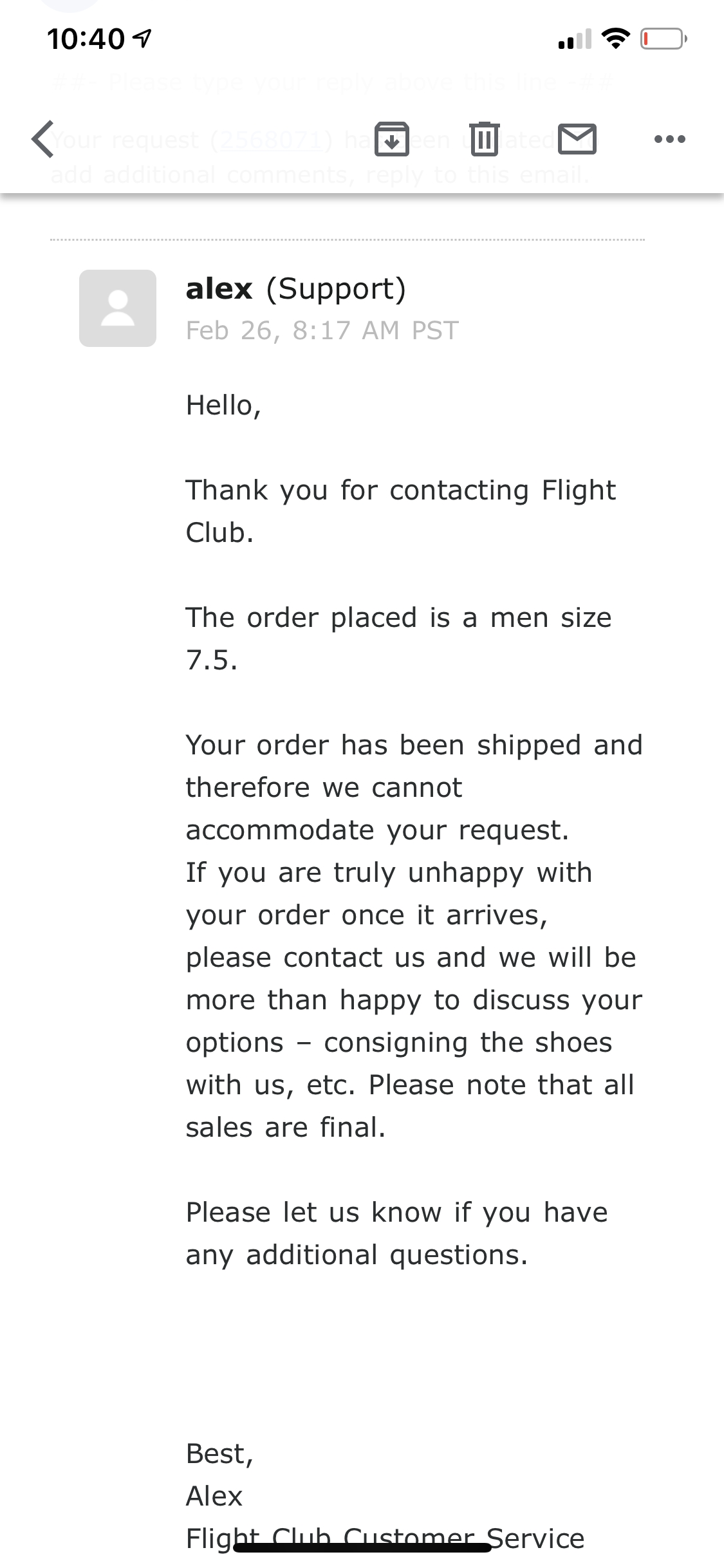The image depicts a cell phone screen displaying a support email. The screen's top banner shows the current time as 10:40 AM, accompanied by a small arrow icon pointing to the right. Adjacent to these elements on the right side of the screen are standard phone icons, including the signal strength indicator and battery power level. 

Below this banner, several icons are visible: a trash can for deleting messages, an envelope for emails, three vertical dots indicating a menu, and a downward-pointing arrow, possibly for downloading or more options. A chatbot message is present with a small square avatar featuring a face and the name "Alex," labeled as "support" in parentheses, dated February 26th at 8:17 AM PST.

The main content features an email response from Flight Club’s customer service, signed by Alex. The email addresses a customer's inquiry about an order for a men's size 7.5 shoe, stating that the order has already been shipped and thus cannot be modified. However, it offers further assistance if the customer is unhappy, mentioning that all sales are final. The email closes with an invitation to reach out for additional questions and is marked by a signature line at the bottom.